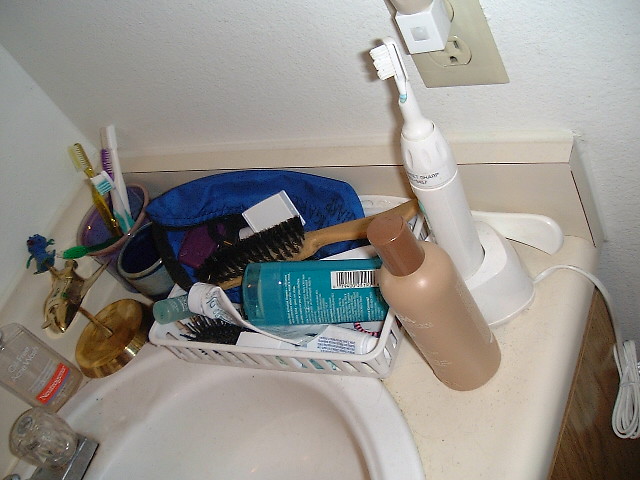This image captures a detailed view of a bathroom sink in the corner of a wall, showcasing a variety of grooming and hygiene items. The sink itself is white porcelain, partially visible at the bottom-left with a clear plastic faucet handle. The countertop is cream-colored, bordered by a white wall. Above the sink, an off-white outlet hosts a white nightlight.

On the counter, there's a white basket containing a mix of items including toothpaste, several hairbrushes with black bristles, deodorant, and a blue bag. In front of the basket sits an electric toothbrush in its charging station, adjacent to a brown cylindrical bottle with a dark brown cap, possibly soap or lotion. Additional toiletries such as skin lotions, acne wash (Neutrogena), and a make-up pad are scattered around.

Towards the back, a cup holds multiple toothbrushes in various colors including green, yellow, purple, and white, indicating usage by multiple individuals. Next to this cup is a small decorative statue resembling a dolphin or possibly an airplane, adding a touch of whimsy to the scene. The countertop provides a comprehensive snapshot of everyday personal care items neatly organized yet naturally arranged.